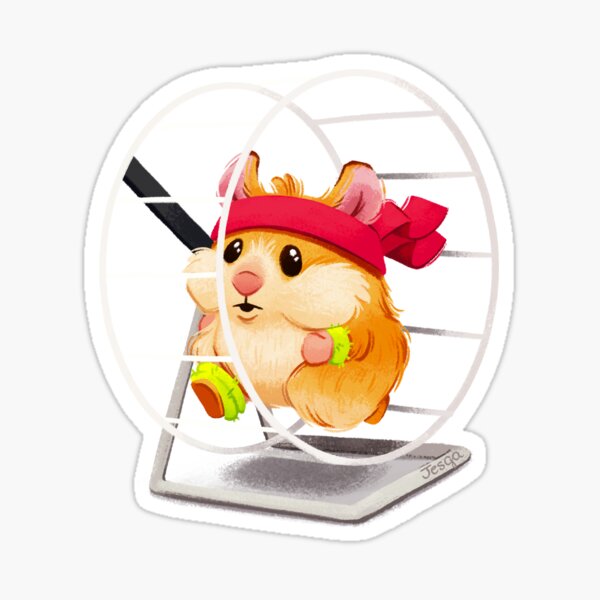This detailed, cartoon-like watercolor drawing features a playful hamster energetically running inside a white and grey hamster wheel, resembling a treadmill with its visible silver bottom part. The background is a subtle light grey, while the center of the image remains white, emphasizing the hamster's lively motion. The adorable hamster, with its charming pink nose and round black eyes, has a distinct orangish-yellowish-brown body complemented by chubby tan cheeks and a white belly. It sports a red headband, with its pink ears protruding through, and green wristbands on its front paws and one of its legs. Adding a dash of flair, the hamster also wears a red bandana tied around its neck, with its loose ends fluttering behind as it runs. The overall effect is a joyful and animated depiction of a hamster engrossed in its workout, bringing a sense of fun and energy to the scene.